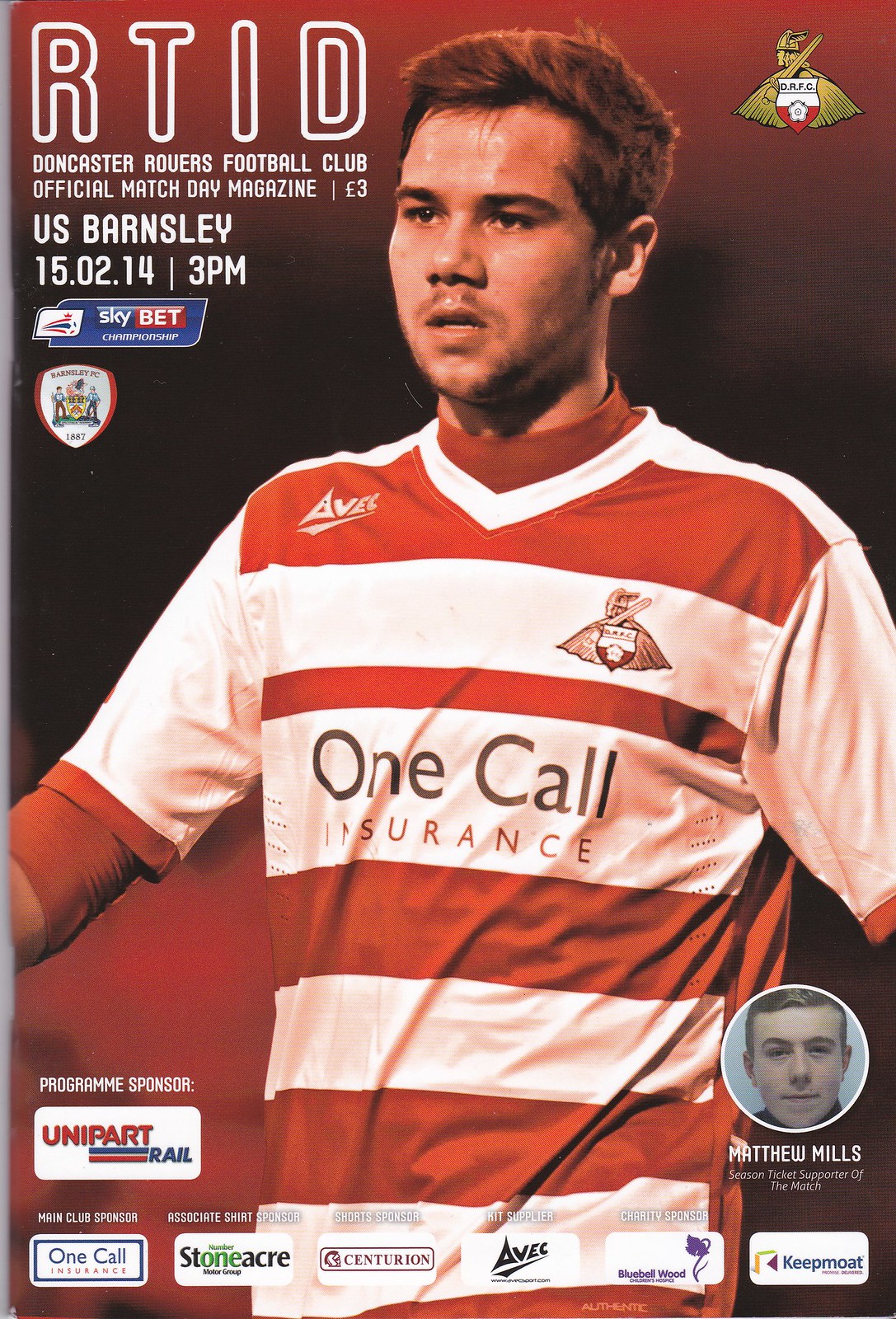This is a color image of the front cover of a matchday program for a soccer (football) match. The cover prominently features a male football player wearing a red and black striped kit with the One Call Insurance logo. The background is a mix of red and black. In the top left corner, the initials "RTID" are displayed, followed by "Doncaster Rovers Football Club". Below, it reads "Official Match Day Magazine, three pounds" and specifies the match details as "U.S. Barnsley, 15-02-14, 3 p.m." The program sponsor is listed as Unipart Rail. Other sponsors mentioned at the bottom include Stoneacre, Centurion, and Keep Moat. Located in the bottom left corner is the Skybet logo, while the top right features the Doncaster Rovers Football Club (DRFC) shield, depicting a Viking with a helmet and sword. Finally, the bottom right corner includes a profile picture of Matthew Mills labeled as "season ticket supporter of the match".